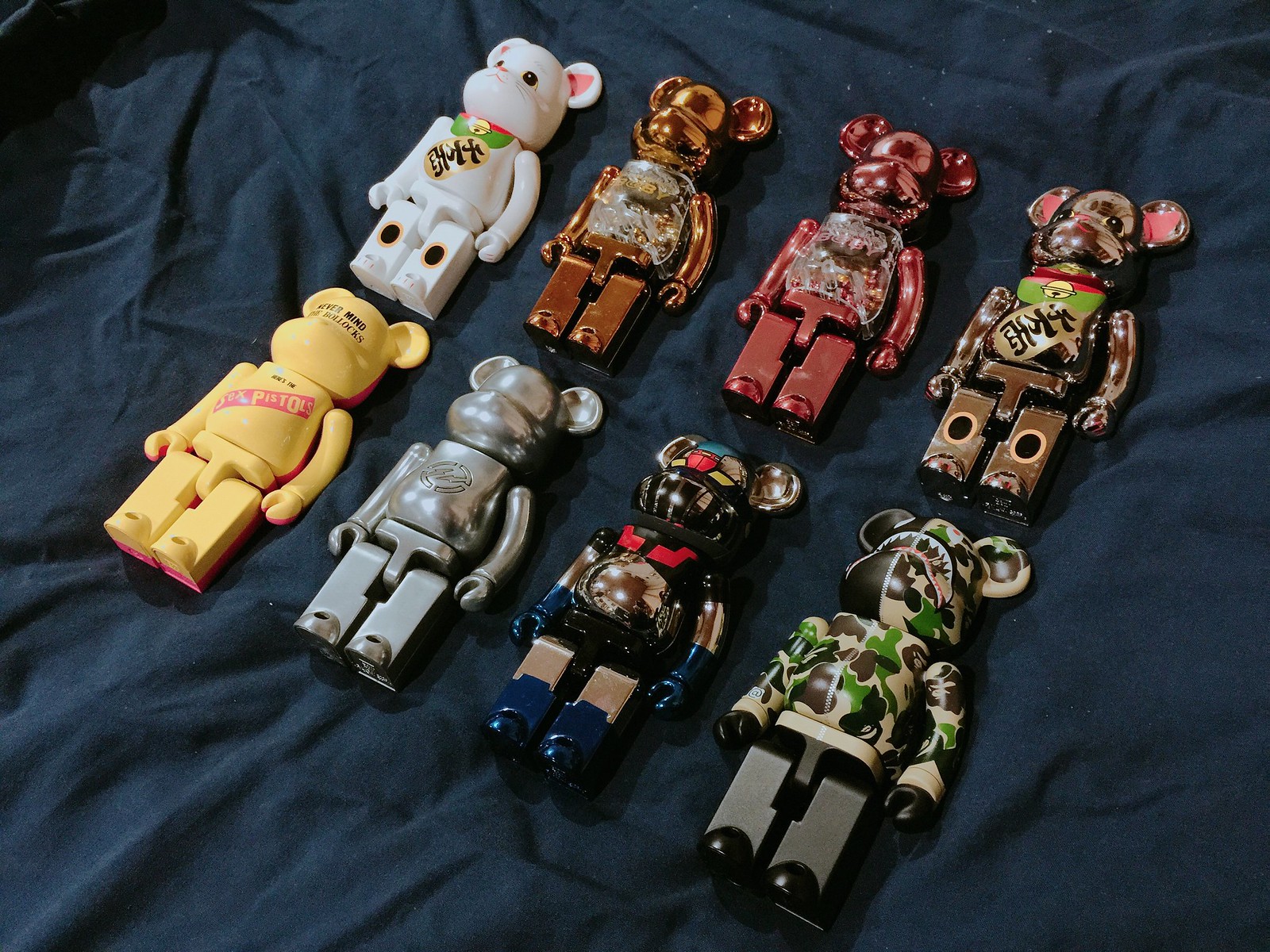The image features eight miniature teddy bear-like figurines arranged neatly in two rows of four on a dark blue, wrinkled comforter that serves as the backdrop. Each figurine, approximately three inches tall, shares a similar shape but differs in color and pattern. Starting from the top left, the first bear is white with pink ears and a small gold patch on its belly. Next to it, is a bronze bear, followed by an iridescent shiny red one. The fourth in the top row is mainly brown with pink ears and has gold and red patterns with calligraphy on its chest. 

In the bottom row, the bears start with a yellow one that has a pink rectangle with some text on it. The next is an all-silver bear, followed by a unique one that's black and red with blue gloves and a mix of red, yellow, and blue on its face. The last bear in the bottom row sports a distinctive camouflage print long sleeve top and hat area, integrated into its teddy bear shape with a half-and-half face design. Some bears feature Asian writing and other intricate designs, adding to their varied and detailed appearances.